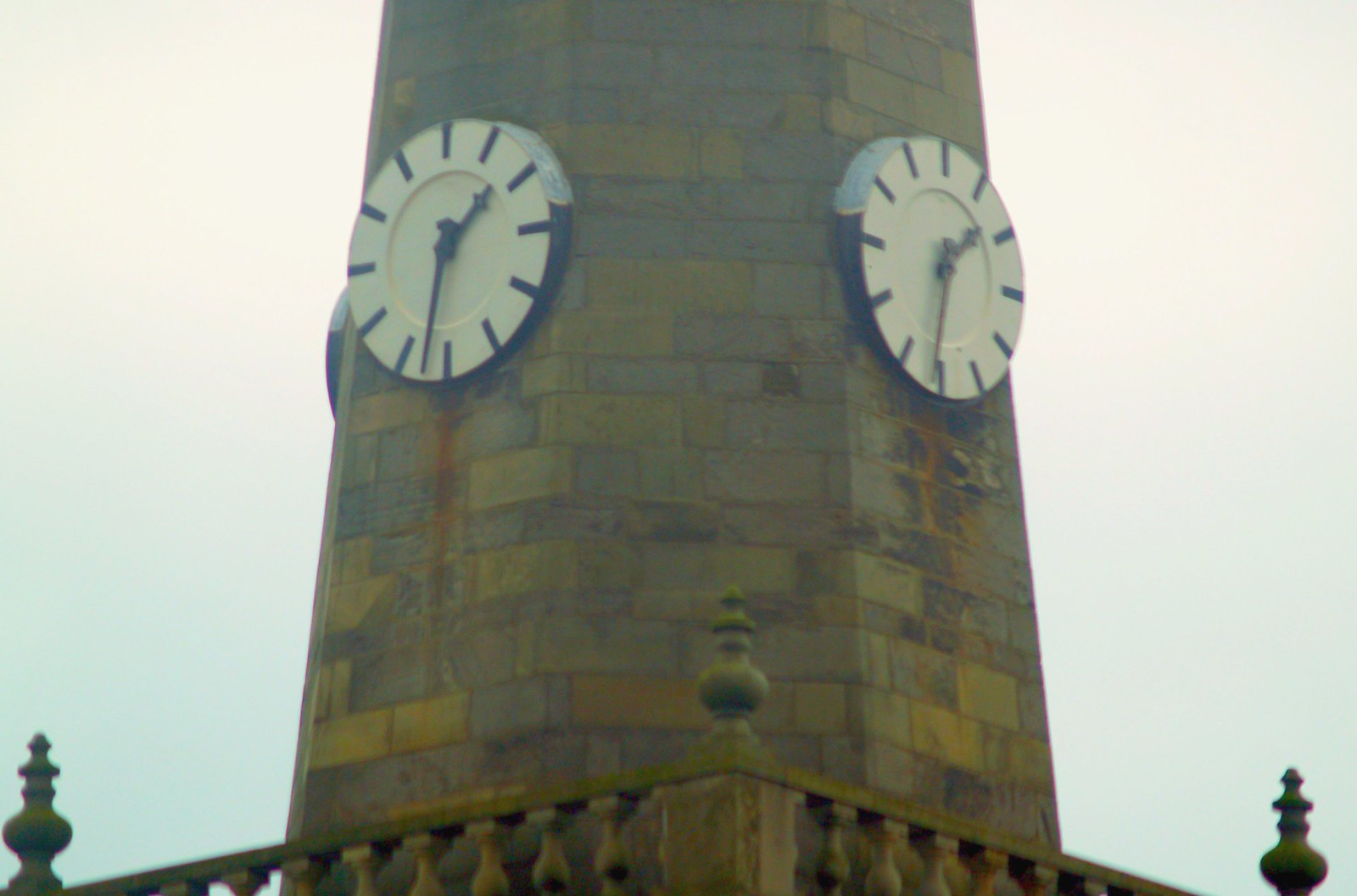The image depicts the top portion of a tall brick tower, likely part of a church or clock tower. The brickwork varies in color, featuring hues of gray, beige, blue, green, red, and brown, giving it a textured appearance. Surrounding the top is a concrete or golden-brown balcony, possibly serving as a lookout point. The tower features multiple clocks; two prominent white clock faces with black outlines and dashes for numbers are visible, both showing a time slightly past 1:30. A third clock face can be partially seen around the corner, suggesting there may be a total of four clocks on the tower to display the time in all directions. The structure appears weathered, with signs of rust near the clocks' edges.